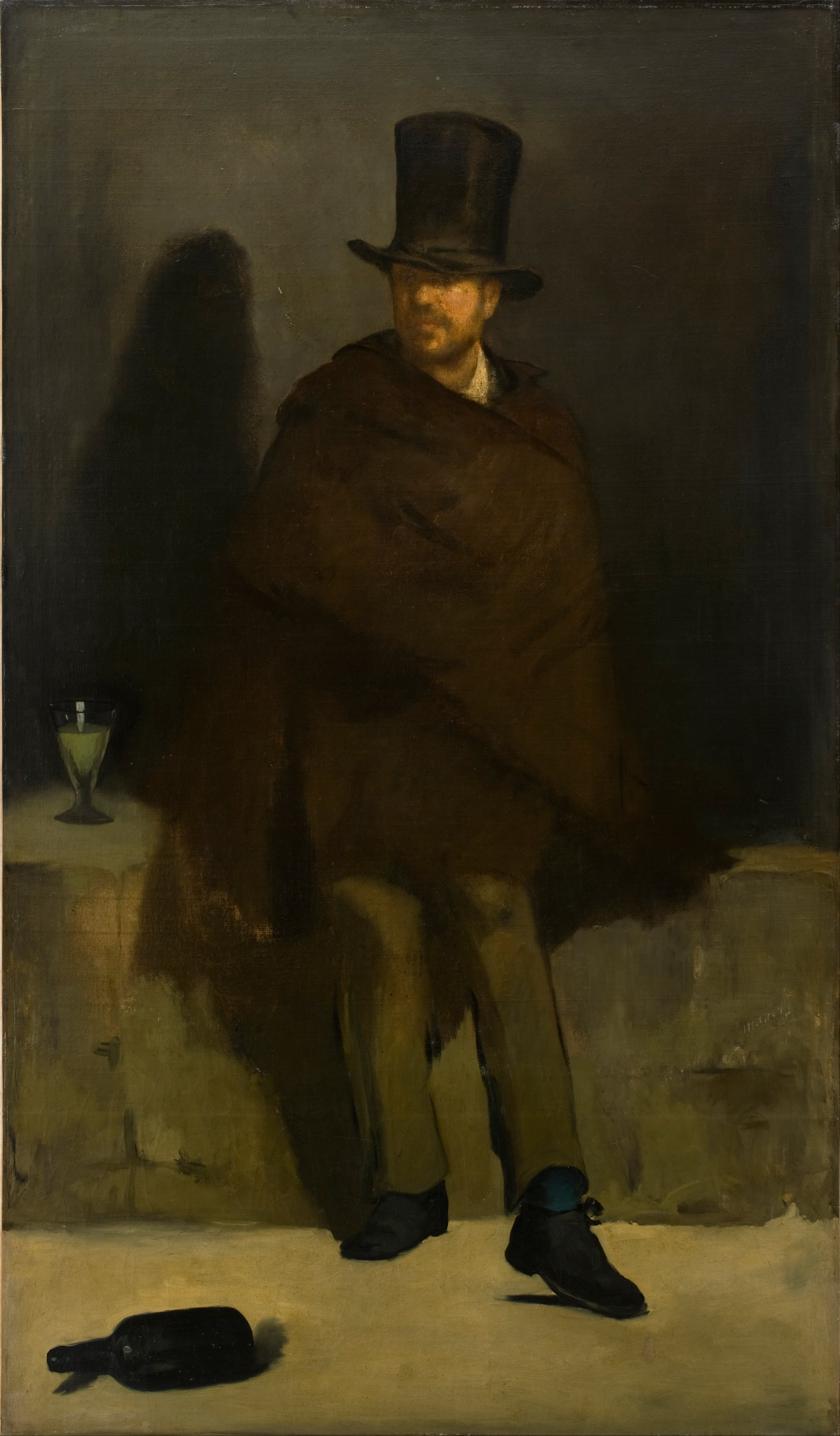This painting features a long, rectangular canvas that captures a solitary man standing against a short stone wall. The man, who exudes the aura of a chimney sweep, is cloaked in a chocolate-brown, blanket-like wrapping over his upper body and wears dark brown trousers paired with black ankle boots. His ensemble is completed with a tall black top hat. He has a neatly trimmed beard and a stubble mustache, lending a rugged charm to his fair complexion. 

He appears to be leaning slightly against the wall, with one foot extended out in front, showcasing a dark blue sock. To his right (and the viewer's left), a glass containing a green liquid rests on the ledge, while a black liquor bottle, perhaps a wine bottle, lies on the ground in front of him. The background is dominated by a dark, grayish-black wall, tinged with shades of green, casting a shadow that mirrors his figure and adds depth to the scene. The man gazes off-camera, lost in thought as if on a contemplative break.